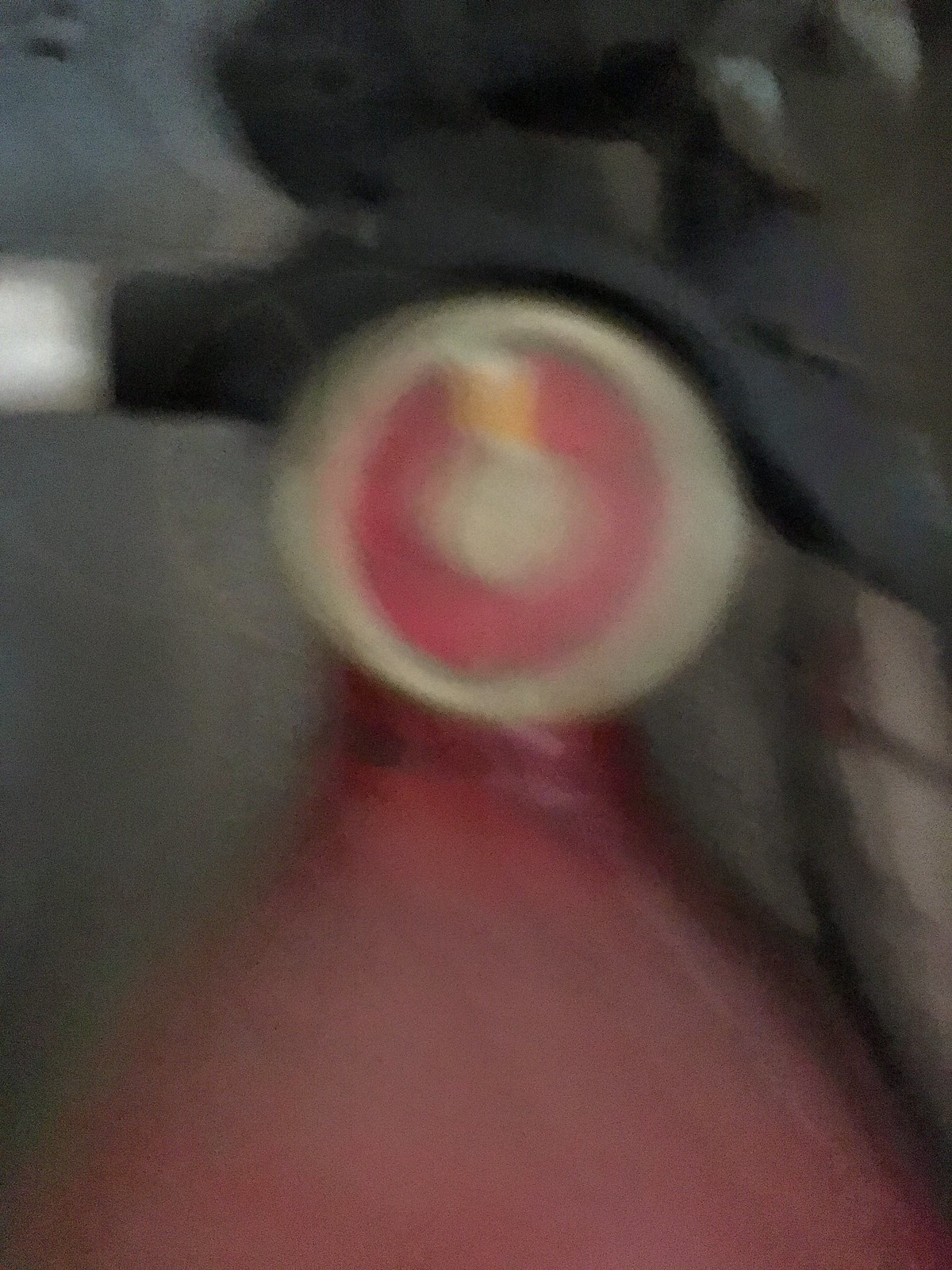A close-up photograph captures a blurred image of a red valve or cap set against a grey backdrop. The photo is taken in motion with inadequate lighting, obscuring fine details and leaving the viewer with an indistinct impression. The red cap appears to be part of a larger red object, potentially a fire hydrant or an air pressure tank, identifiable by what seems to be a nozzle indicator. Due to the proximity of the shot and lack of clear perspective, it's challenging to discern the exact size or scale of the object.